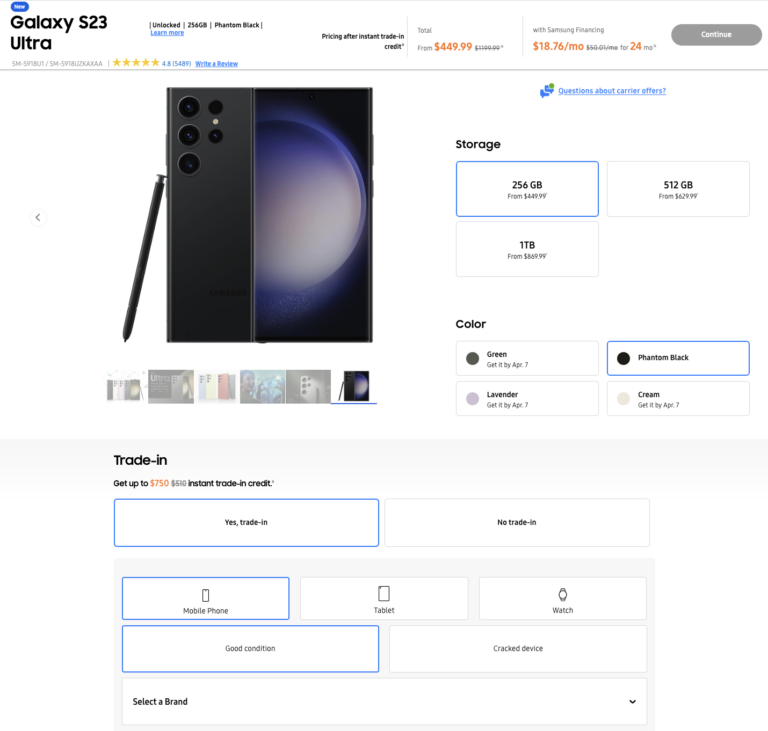The image depicts a detailed screenshot of an online store page for the Galaxy S23 Ultra. In the upper left-hand corner, a blue label marked "New" is prominently displayed. The phone is an unlocked model with 256 GB of internal storage and is shown in the Phantom Black color option. A blue "Learn More" button is visible alongside the pricing information, which lists the phone at $449.99 after an instant trade-in credit. For those opting to finance via Samsung, the monthly cost is $18.76 over 24 months.

The main section of the page features a large, clear image of the Galaxy S23 Ultra, highlighting its key features including three large cameras, two additional smaller cameras, and a stylus. To the right of this image, the selected storage option of 256 GB is displayed, with additional options of 512 GB and 1 TB available for selection.

Below the main image, there is a series of smaller thumbnail images of the phone, allowing for a closer look when clicked. Color options for the device include green, phantom black, lavender, and cream. 

At the bottom of the page, a Trade-In menu appears. The trade-in section is highlighted in blue, indicating an active trade-in selection, while an option for "No Trade-In" is available but not selected. The trade-in details specify a mobile phone in good condition, though the specific brand has not yet been chosen.

Overall, the screenshot illustrates the process of purchasing a Galaxy S23 Ultra with an active trade-in option.